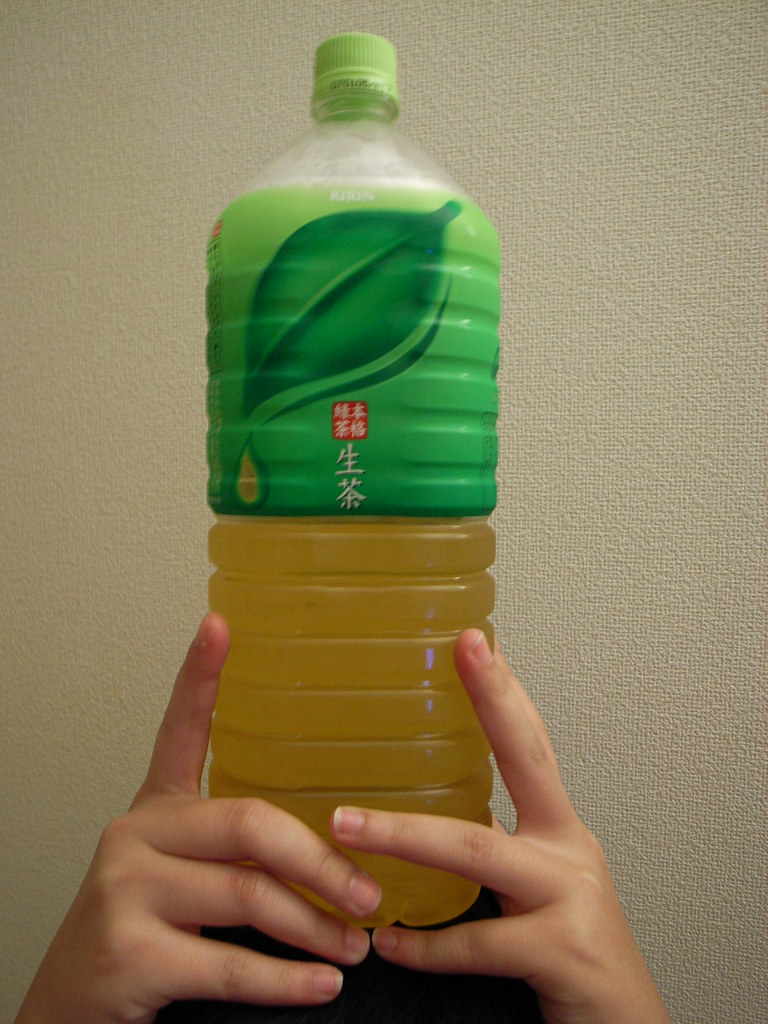In this close-up photograph, a person, whose identity is obscured, holds a large bottle of what appears to be green tea against a textured white wall. The bottle is adorned with a green cap, and the label, also green, prominently features an illustration of a leaf. A drop of the tan-colored drink clings to the bottle, hinting at the liquid's hue. Intriguing Chinese symbols in a red square, along with additional characters beneath, embellish the label. Although some white lettering is visible, it is partially obscured by the light reflecting off the bottle. The entire scene emanates a sense of freshness and simplicity.